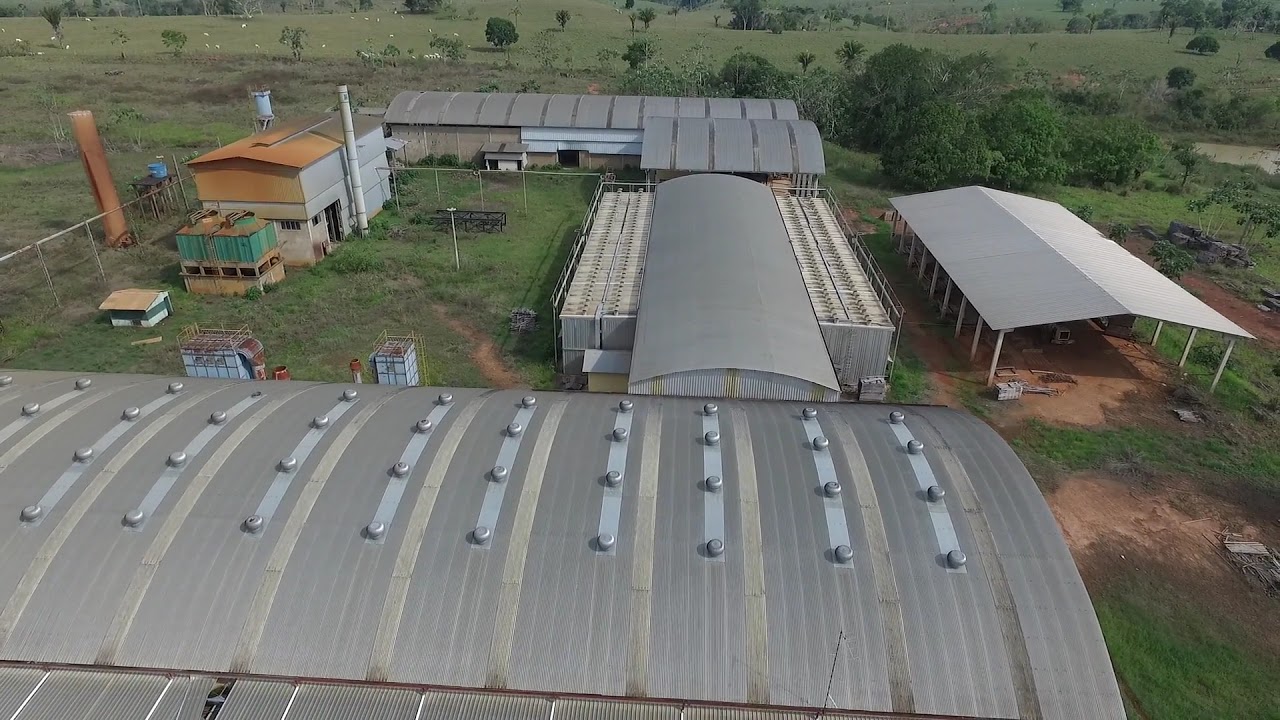This aerial photograph captures a picturesque countryside farm bathed in daylight. The image is framed horizontally, taken from an elevated vantage point, possibly from a rooftop. Dominating the foreground is a large silver building with distinctive blue vertical stripes and small knobs along each stripe. This building, possibly a greenhouse or chicken coop, lies at a right angle to another attached gray building, creating a central right-angle structure. This central structure forms the focal point from which other elements radiate.

To the right of this central angle, a substantial grayish-white awning extends, large enough to shelter multiple vehicles or RVs, providing a practical covered space. In the middle background, there is another gray building, further contributing to the utilitarian aesthetic of the farm structures. To the left of the right-angle junction, another smaller building stands out with a rust-colored roof and visible wires, adding a quaint touch to the setting.

The farm is interspersed with greenery; lush green grass, scattered bushes, and mature trees frame the scene, enhancing the rural charm. Towards the top left, additional sheds or garages and some fencing details are faintly visible, suggesting ample storage and delineated spaces for farming activities. The distant backdrop of trees further accentuates the serene, bucolic atmosphere of this countryside farm.